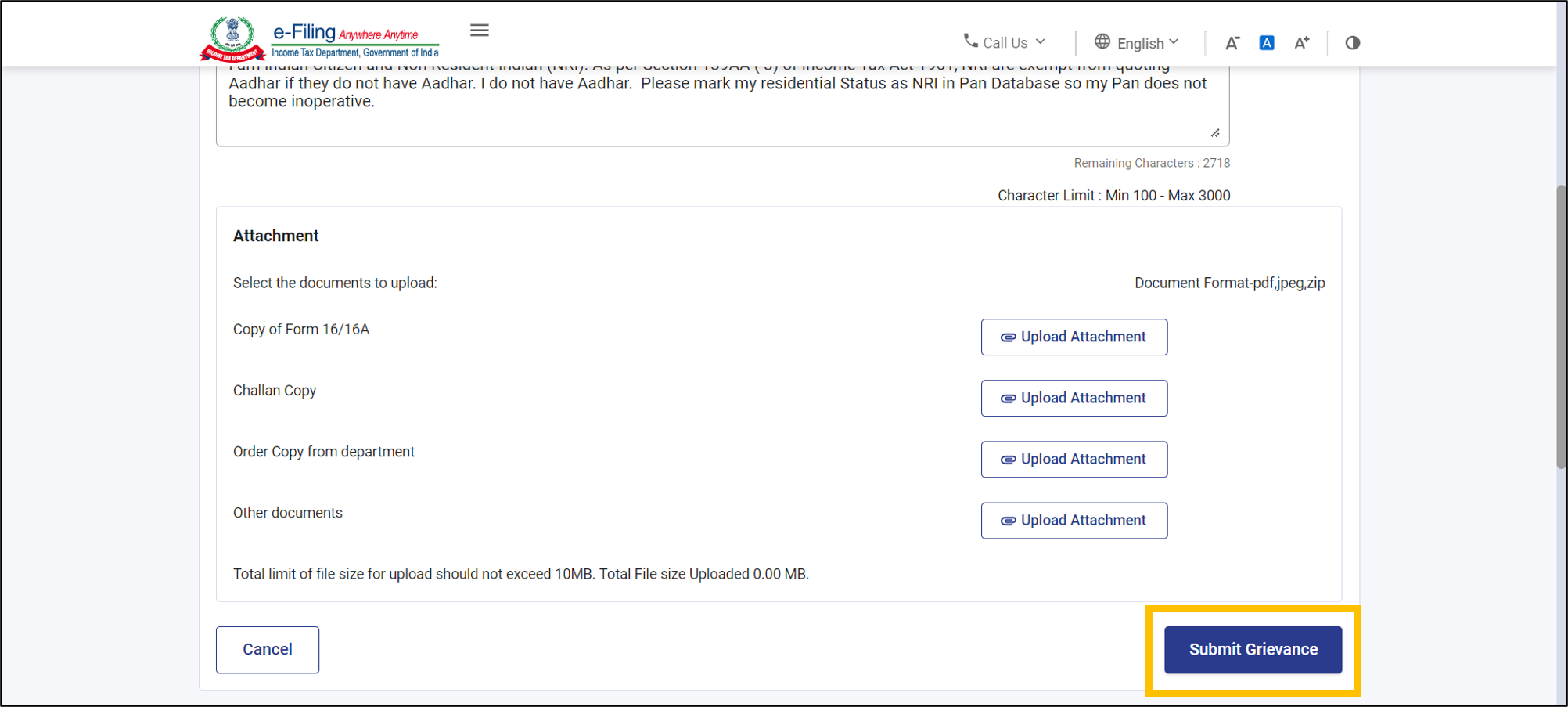The image depicts a website interface designed for electronic filing, prominently titled "E-Filing" followed by two additional, partially blurred words that both appear to start with the letter 'A'. On the left side, an icon presumably symbolizing e-filing is present, adorned with a banner containing some text. To the right, the interface features a phone icon labeled "Call Us" accompanied by a drop-down arrow. Further right, a line separates this section from the next which includes a globe icon and an associated drop-down arrow representing language selection. Following a second line separator, there is a visual element with three large 'A's and a circle that's half black and half white, likely denoting text size or color settings.

Below this, a partially visible paragraph body is truncated, showing only the last two sentences. Adjacent to it, text states "Character limit: minimum 100, maximum 3,000," located near the left side of the section. Below this informational text, there is a square section labeled "Attachment," featuring six rows, each with an "Upload Attachment" button.

At the bottom of the interface, on the left side, there is a "Cancel" button; on the right side, a "Submit Grievance" button is displayed—it is blue with a distinctive yellow outline.